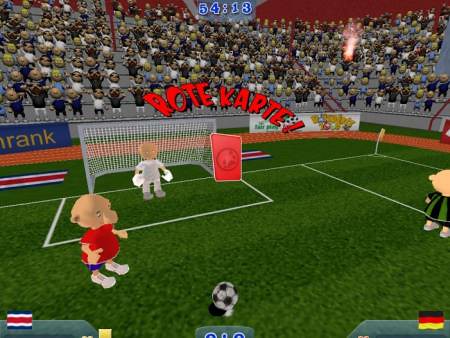In this rectangular image, we are immersed in a vibrant scene from a video game that depicts an intense moment on a soccer field. Dominating the lower center of the image is a soccer ball, seemingly poised for action. To the left, a soccer player dressed in a red shirt, blue shorts, and white shoes appears ready to make a move. Guarding the goal is another player, clad entirely in white, standing alert and prepared to defend. Near the center right, an umpire in a distinct blue and green vertically striped shirt closely observes the play. The stands are densely packed with miniature spectators, their excitement palpable even in their tiny form. Adding a touch of branding to the scene, the word "Cartier" is prominently displayed in bold red block print to the right of the goal. The overall energy of the image captures the dynamic and thrilling atmosphere of a high-stakes soccer match.